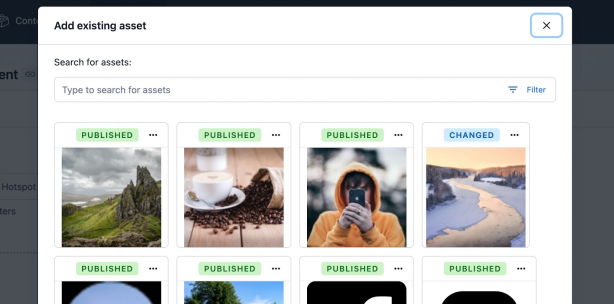The image showcases a grayed-out website in the background with a prominently displayed "Add Existing Asset" pop-up window in the foreground, which is white. In the top right corner of the pop-up, there is a light gray 'X' button outlined in blue and filled with white. On the top left, the heading "Add Existing Asset" is written in black font. Below the heading, a thin gray line separates the top section from the search interface. Beneath this line, in a smaller black font, is the instruction "Search for assets", followed by a search bar that contains the placeholder text "Type to search for assets." A filter button is positioned on the right side of the search bar.

The body of the pop-up displays a series of thumbnail images arranged in a grid. From left to right, the visible images include a green mountainside, a cup of coffee with coffee beans spilling out to the right, a boy in an orange sweatshirt holding a phone up to his face, and a snowy landscape with a river running through the middle. Below the thumbnails, additional images are partly visible but cut off by the edge of the picture. Above the first three visible thumbnails, there are green "Published" buttons with dark green text, each accompanied by ellipses on their right. The thumbnail of the snowy landscape has a blue "Changed" button with blue text.